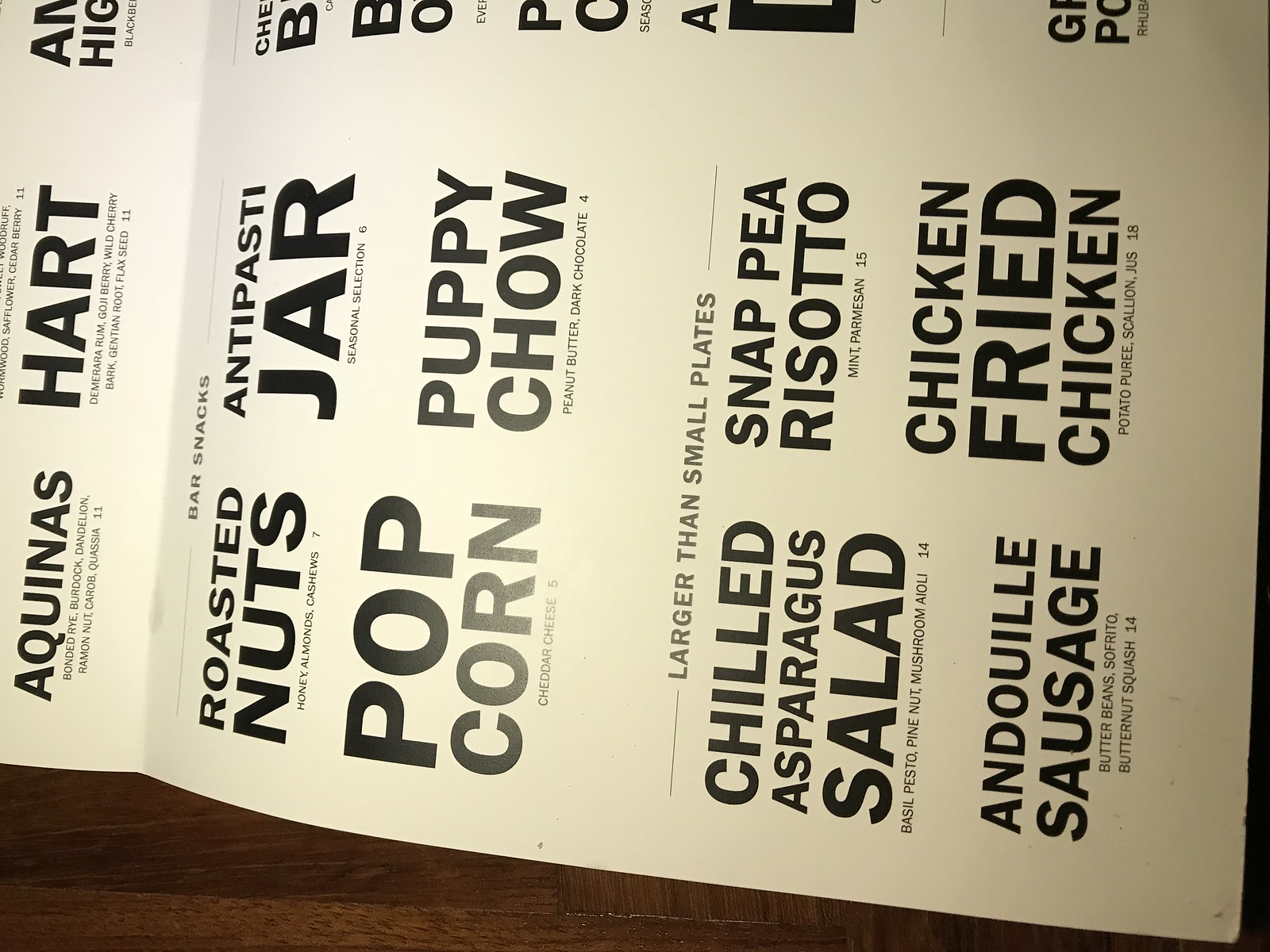A detailed close-up shot of a menu printed on white paper, captured sideways due to a quarter turn to the left. The menu, simply printed, showcases "Aquinas" at the top in bold black letters, followed by "Heart" in the middle, with another unreadable row beneath it. Under this, the text "Bar Snacks" appears in dark gray, listing items such as Roasted Nuts, Popcorn, Antipasti Jar, and Puppy Chow in bold black print. The next section, titled "Larger Than Small Plates", presents options like Chilled Asparagus Salad, Andouille Sausage, Snap Pea Risotto, and Chicken Fried Chicken, all also in bold black print. Evident creases suggest the menu had been folded in half and then opened. It rests face-up on a glossy brown wooden table, partially visible at the bottom of the image. A bright overhead light shines on the menu, creating a noticeable reflection in the middle.